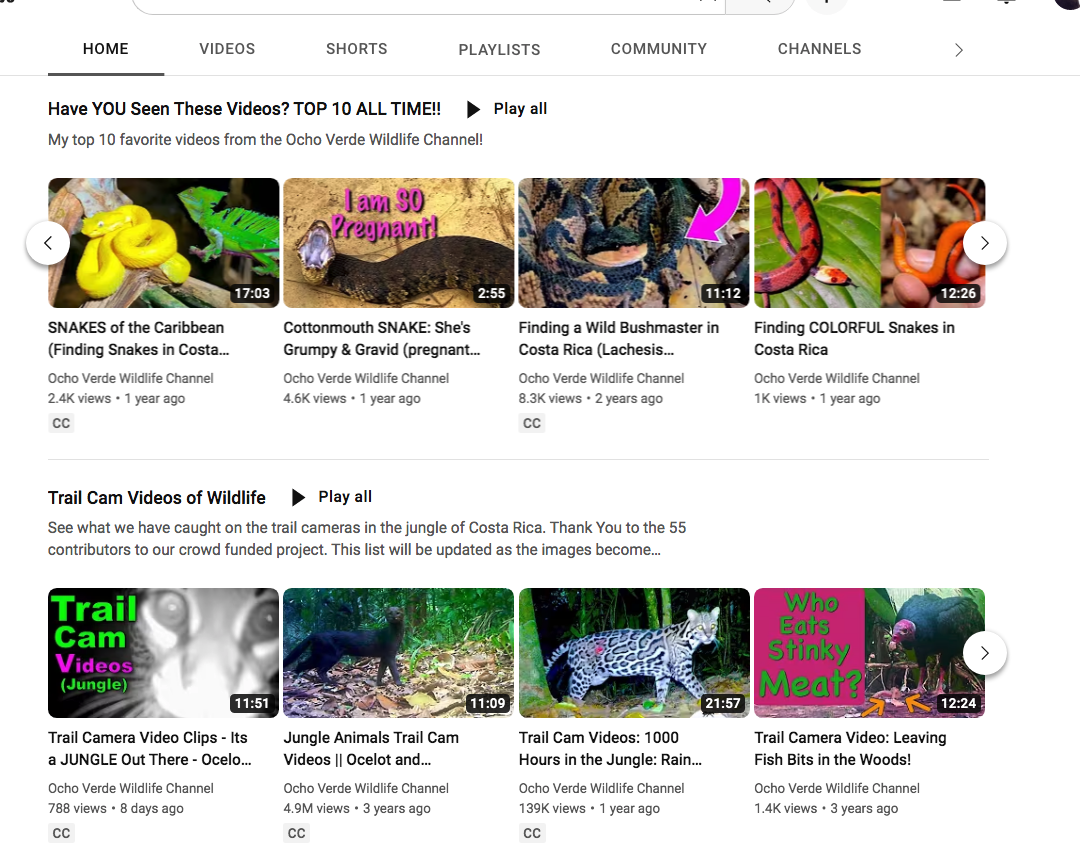Here's a detailed and cleaned-up descriptive caption based on the provided voice transcription:

---

"Welcome to the Playlist Chameleon Channel! In this video, I present my top 10 favorite videos from the Ocho Verde Wildlife Channel—renowned for its captivating wildlife footage from the Caribbean and Costa Rica. 

1. Featured prominently is a video of a striking yellow snake with a green iguana in the background.
2. The exciting "Snakes in the Caribbean" series showcases the diversity of serpentine life in the region.
3. Our "Finding Snakes in Costa Rica" segment highlights a grumpy and gravid Cottonmouth snake, recorded a year ago with an impressive 4,000 views.
4. One of the fan favorites, "Finding a Wild Bush Monster in Costa Rica," uncovers the vibrant reptiles of the lush jungles.
5. Another thrilling entry, "Finding Colorful Snakes in Costa Rica," has garnered enthusiastic audience engagement.
6. Our trail cam compilation shows the extraordinary wildlife activity captured by our jungle cameras, thanks to 335 contributors to this crowdfunded endeavor.
7. Regularly updated with fresh footage, our trail cam series reveals intimate glimpses into the jungle's natural residents.
8. Recently, a trail cam video posted just 8 days ago has already drawn considerable attention with thousands of views.
9. The immensely popular "1,000 Hours in the Jungle" video has achieved 1.39 million views within a year.
10. Lastly, "Who Eats Stinky Meat?"—a trail cam video featuring wildlife attracted to fish bait—has captured 1.4 million views over three years.

Join us as we delve deep into the wonders of Ocho Verde, witnessing the vibrant and often hidden lives of Costa Rica's wildlife through the lens of our trail cameras."

---

This refined caption provides a coherent and engaging summary of the video content, enhancing the viewer's understanding and interest.